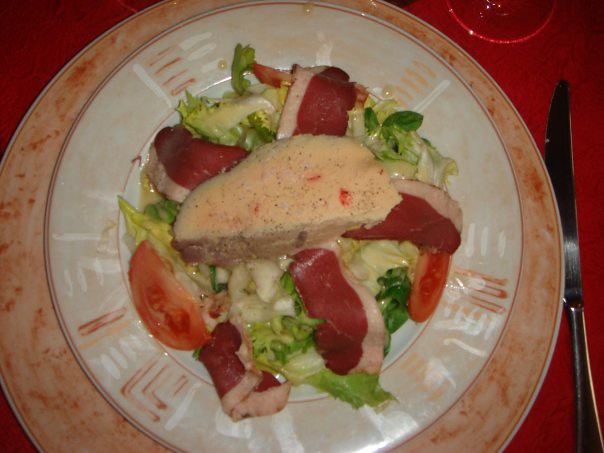This photograph captures a somewhat dark and poorly lit image of a meal on a plate, making some details hard to distinguish with clarity. The food appears to be a green salad featuring iceberg lettuce, tomato wedges, and possible strips of bacon or another type of meat, with hints of onion. A thick, spongy piece of bread sits atop the salad, which is garnished with some kind of salad dressing. The food is presented on a small, white circular plate with an intricate orange or peach tribal border design. This white plate rests on a larger orange plate with various shades and patterns of orange. The plates are placed on a red surface, possibly a table or tablecloth. In the upper right corner of the image, part of a drinking glass is visible, along with a silver table knife positioned to the right of the plates, completing the scene.